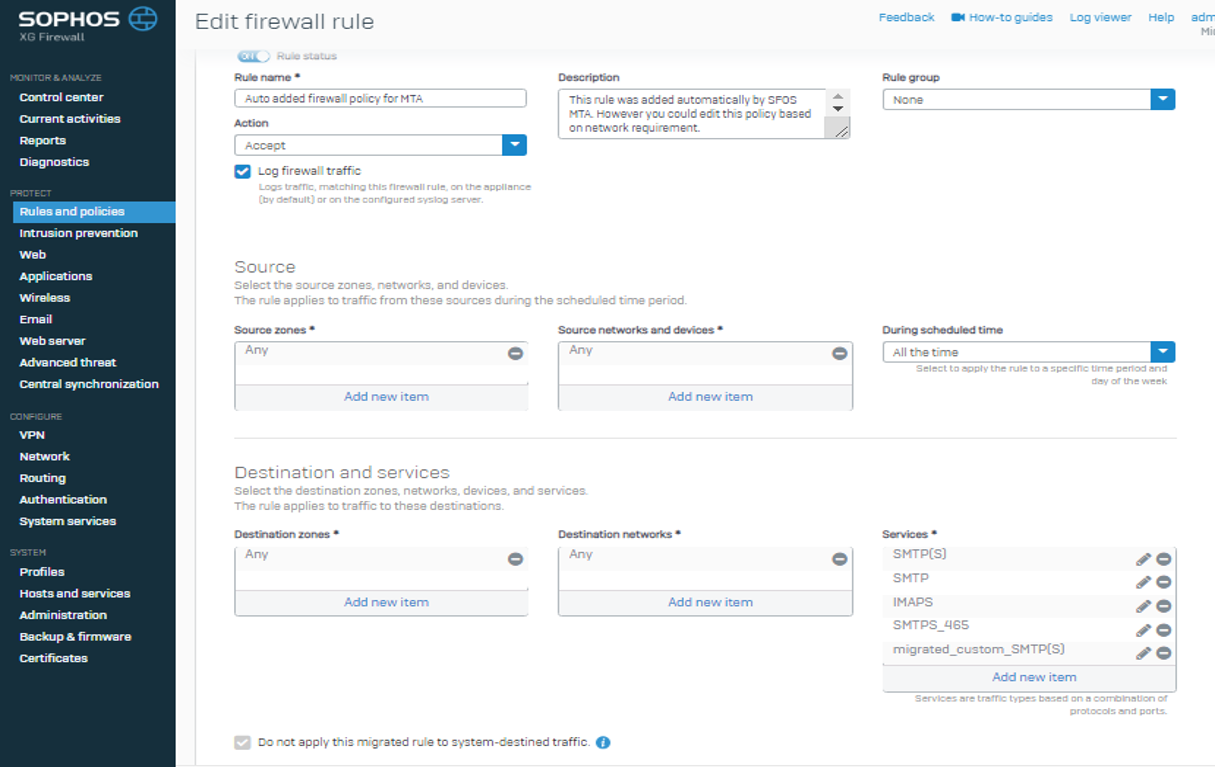This image features a screenshot of an application or program, presented in a landscape orientation with no defined borders. On the left side of the image is a vertical column with a dark blue background, prominently displaying the word "Sophos" in white lettering at the top, alongside a blue circular icon. Beneath the icon, in smaller font, is the text "Add Firewall." 

This column contains several headers and subcategories, with the headers in gray and the subcategories in white. The headers include "Monitor and Analyze," "Protect," "Composure," and "System." Under the "Protect" header, the subcategory "Rules and Policies" is selected, indicated by a light blue box with white font.

To the right of this column, a gray header labeled "Edit Firewall Rule" in black font spans the top of the main section. Nearby, a series of selectable blue options are arranged horizontally, offering choices such as "Feedback," "How-To Guides," "Log Viewer," and "Help." 

Below this header, the interface features a toggle button for "Rule Status," which is currently set to the right and highlighted with blue lettering. Beneath this are multiple text boxes, suggesting input fields likely used for setting parameters or filters, perhaps for configuring specific firewall rules or policies. The overall layout implies the user is engaged in programming or filtering rules within a firewall configuration tool.